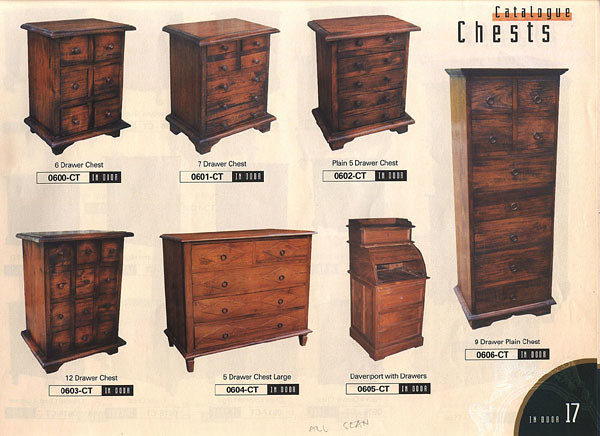This full-color photograph captures a catalog page, numbered 17, advertising various chests of drawers. The background is a pale beige, giving prominence to the seven dark brown chests displayed. Each chest is distinctly labeled: a traditional seven-drawer chest featuring three larger drawers at the bottom and four smaller ones at the top, a compact six-drawer chest with very small drawers, a plain five-drawer chest, and a large five-drawer chest suitable for a bedroom dresser. There is also a towering twelve-drawer chest with square drawers, and a very tall nine-drawer plain chest, which has four square drawers at the top and elongated ones below. Additionally, a Davenport with drawers, resembling a roll-top desk, is featured. The page prominently features the words "Catalog Chests" at the top right.